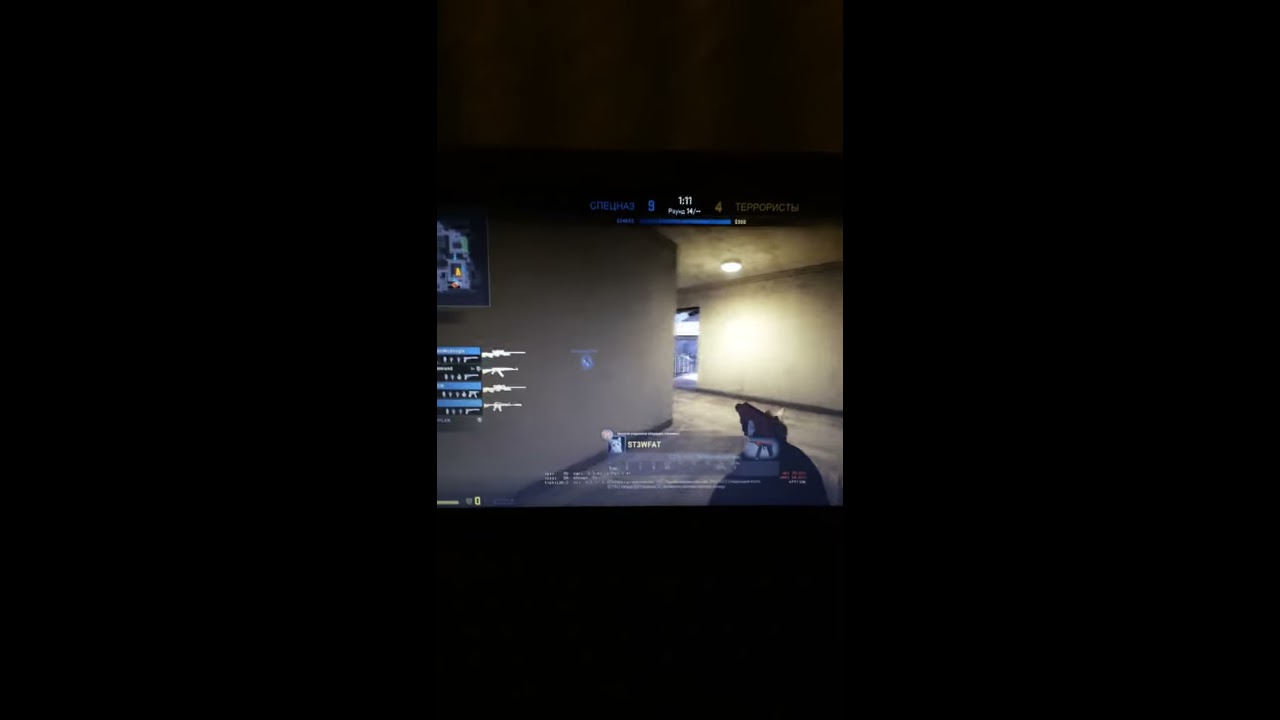This image is a still shot from a first-person shooter video game framed within a very thick black border, making the actual picture quite small against the surrounding black space. The player's perspective is that of going down a curved, dimly-lit hallway which seems to be adorned with a light tan or dingy white wall. The hallway appears to have a ceiling light in view and is carpeted. To the right, there’s an intersecting wall, and the hallway veers to the left, revealing an open area or another doorway as it curves. In the lower-right corner of the screen, there's a gloved hand holding a gun. The upper left of the image shows a picture of a white building hanging on the hallway wall. Text overlays are visible, featuring a progress bar at the top and options for selecting from four different weapons at the bottom left of the screen. In the forefront, the numbers nine and four appear as part of the game interface.